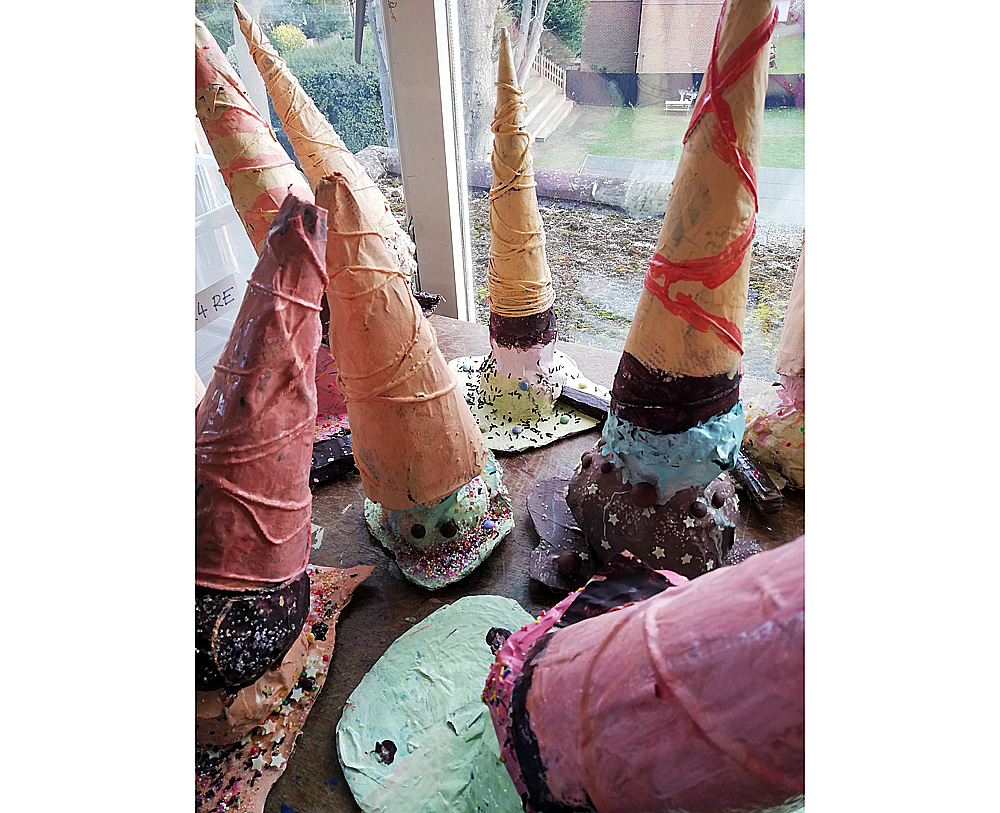A highly detailed photograph depicts a whimsical collection of seven iced cake ball cupcakes, creatively designed to resemble towering ice cream cone hats. Each confection is perched upside down on a windowsill, overlooking a blurred backyard. The cupcakes showcase a variety of vivid colors, including mint-green, chocolate, and sky-blue, some adorned with colorful sprinkles. The imaginative creations feature one to three scoops each, with bases of green, pink, red, or brown. The cones, evoking the shape of elongated witch's hats or dunce caps, appear hand-crafted, possibly as part of a children's art project or a delightful rainy day activity. The playful designs and creative toppings make each cupcake unique, transforming an ordinary treat into a charming and festive visual display.